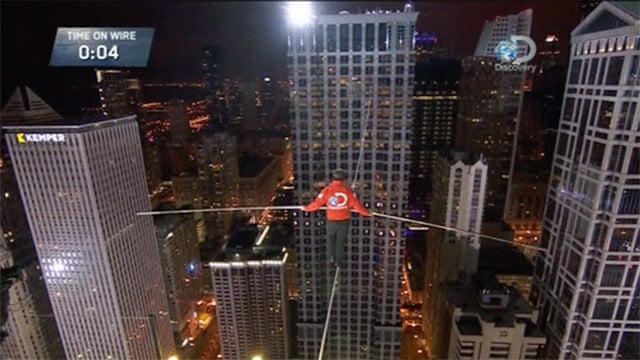This detailed nighttime photograph, originating from the Discovery Channel, captures a dramatic high-wire act set against a backdrop of illuminated city skyscrapers. The image shows a man dressed in black pants and an orange coat bearing the Discovery Channel logo, walking on a tightrope strung between two towering office buildings. The tightrope artist steadies himself with a long balancing pole extending horizontally. The shot, taken from a TV screen, includes a noticeable camera flash in the upper center, adding a reflective glare. In the upper left corner, there's a time box displaying "Time on Wire 004," indicating four seconds have elapsed. The Discovery Channel's logo, depicted as a stylized Earth adjacent to the letter 'D' with "discovery" written below, is prominently visible in the top right. The city's streetlights and the sheer height of the skyscrapers dramatize the depth and scale of this perilous walk.